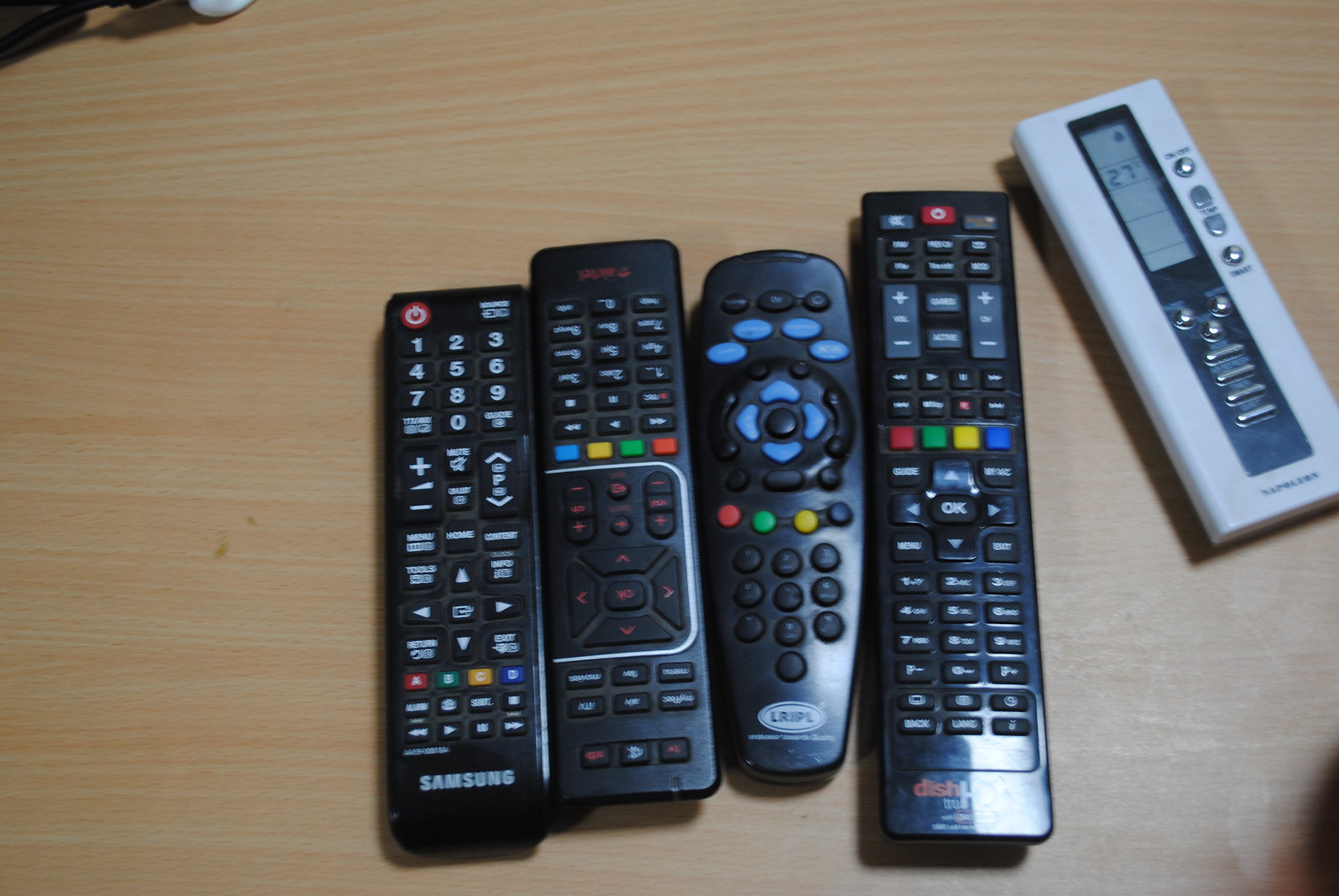The image depicts a scene taken indoors, showcasing a wooden table with a distinct grain texture. On the table lie five remote controls. The four remotes in the center are black and differ in size and brand. Among them, one is visibly made by Samsung, and another by DISH, while the brands of the remaining two are not clear. These remotes are adorned with a colorful array of buttons, including red, green, yellow, blue, and black, with some featuring a standard D-pad in the middle and red power buttons, as well as rows of colored buttons nestled among the primarily black and gray buttons. 

On the far right, there is a distinct handheld device, unlike the others. This device is encased in white or gray plastic, featuring a rectangular strip with silver buttons and an LCD screen displaying the number 27. This device is presumably a type of remote but is clearly not a standard TV remote, possibly serving a different function. 

A light source from behind the camera casts a soft glow onto the table, illuminating the remotes and enhancing the visibility of their various buttons and features.